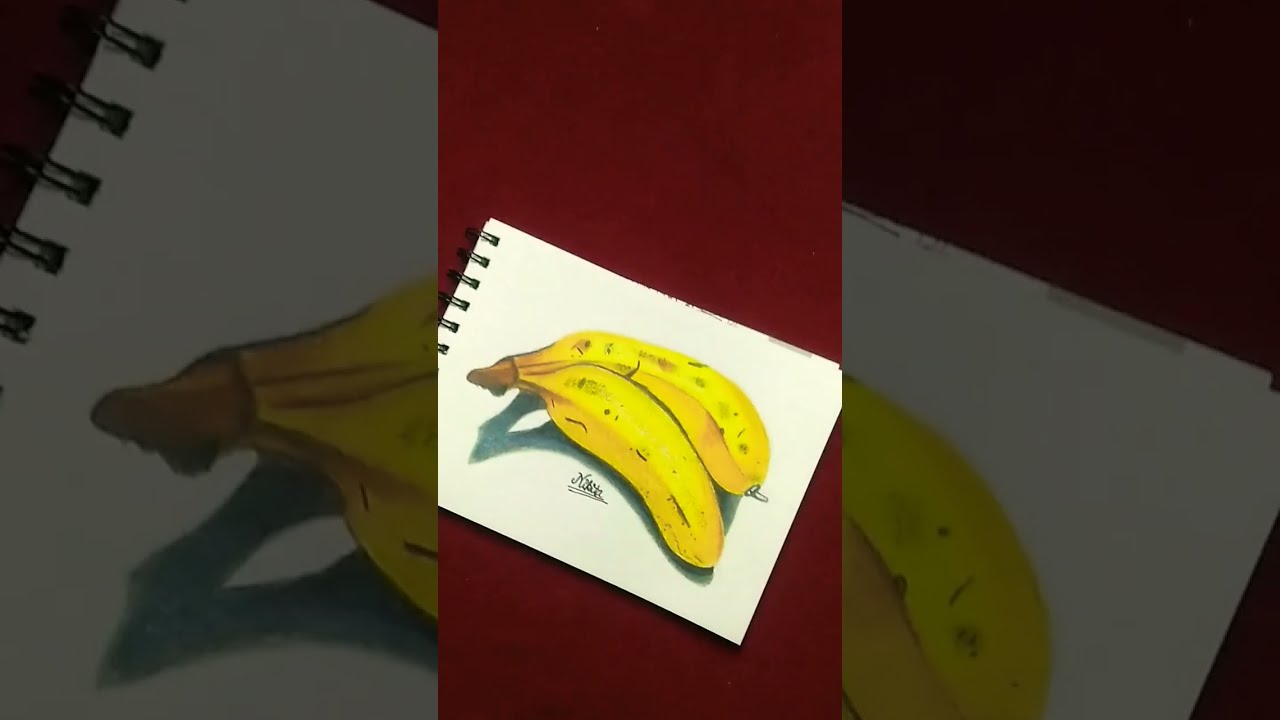The image depicts a notepad with a vertical spiral binding, containing a detailed drawing of two yellow bananas that are connected by the vine. The notepad, with its white pages, showcases the intricate illustration complete with shadows, detailed bruising along the sides, and marks at the top and bottom of the bananas. Below the drawn bananas is the artist's signature. The notepad itself is placed at an angle, with the left edge raised and the lower right side downward, set against a dark red background that encompasses the entire scene.